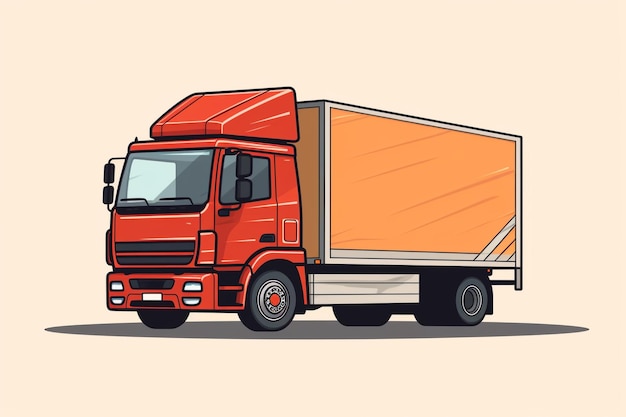The image depicts a detailed, cartoon-style drawing of a delivery truck, positioned facing left and centered against a light pink or beige background, with its dark shadow extending beneath it. The cab of this cab-over style truck is predominantly red and features several distinctive elements: black bars on its blunt front grill, a pair of windshield wipers at the base of the windshield, and double side view mirrors on each side.

The truck has black wheels with prominent red hubcaps on the front wheel. Additionally, notable is a wedge-shaped structure atop the cab, possibly for aerodynamic efficiency or housing equipment. The rectangular cargo compartment in the rear is light brown or tan with a metallic gray or white frame, and includes some protective metal running board extending halfway along its side.

Simplistic in its design, the truck also includes small details like a gas tank door on the side and a straightforward pattern without any text overlays. Its minimalistic look and highlighted features make it the primary focus of the image.